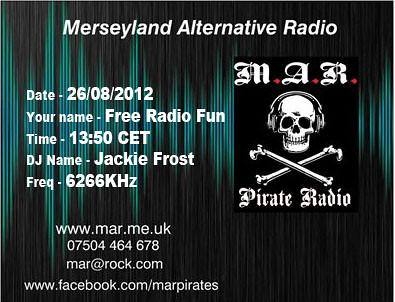The image appears to be an advertisement or informational card designed for social media or website promotion. The background features a combination of bluish-green and black, creating a wave pattern reminiscent of audio lines. At the top, the banner reads "Mercyland Alternative Radio" in white. On the right side, there is a black square with a logo that includes the letters "M.A.R." in an old script, positioned above a skull and crossbones wearing headphones, resembling a Jolly Roger pirate flag. Below the skull and crossbones, the text "Pirate Radio" is prominently displayed in white.

On the left side of the image, there are several labeled sections with information:
- **Date:** 26/08/2012
- **Your Name:** Free Radio Fun Time
- **Time:** 1350 CET
- **DJ Name:** Jackie Frost
- **Frequency:** 6266 kHz

In the bottom left corner, contact details and online resources are listed:
- **Website:** www.mar.me.uk
- **Phone Number:** 07504464678
- **Email:** mar@rock.com
- **Facebook Address:** www.facebook.com/mar.pirates

This comprehensive design effectively conveys the radio station's identity and essential broadcast information.